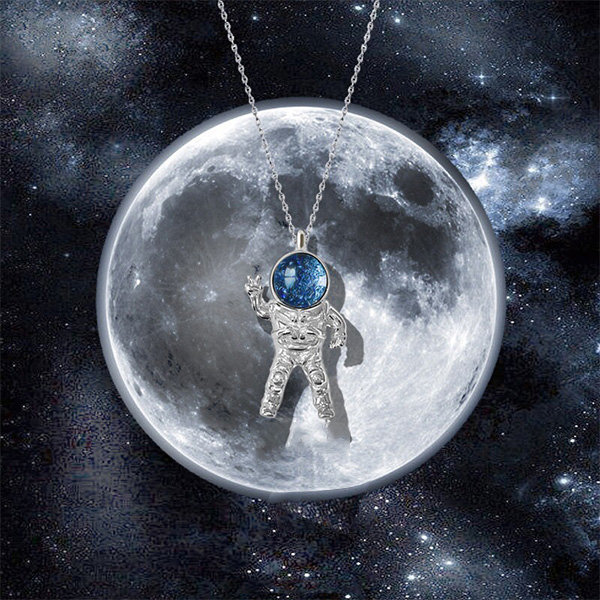The image is a meticulously crafted digital photograph featuring a silver astronaut necklace suspended against a cosmic backdrop. The background showcases a detailed depiction of outer space, with a vast, dark expanse dotted by numerous white stars. Dominating the center of this stellar scene is a large, artistically rendered moon bathed in shades of silver, gray, and white.

Descending from the top of the image, a delicate silver chain holds the pendant—a detailed astronaut figure. The astronaut's body gleams with silver tones, and its right hand is raised in a peaceful gesture, forming a peace sign. Notably, the helmet of the astronaut is a striking blue gemstone, enveloped in a glass casing that adds a sparkling, otherworldly touch to the piece. This intricate necklace appears suspended in front of the moon, emphasizing the celestial theme and creating a visually captivating contrast between the terrestrial piece of jewelry and the vast, infinite night sky dotted with constellations.